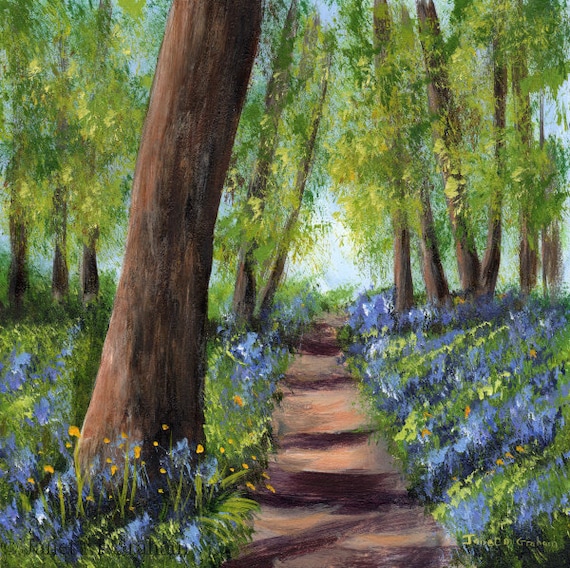This acrylic painting depicts a serene forest scene featuring a cleared path winding off-center to the right, extending from the bottom to about the middle of the frame where it disappears. The heavily impressionistic style suggests it's the work of an amateur artist named Jane Graham, whose name is signed in the lower right corner. The path itself, painted in various shades of brown, is flanked by vibrant grassy fields, dotted with an abundance of blue, yellow, and purple flowers — the latter giving an impression of a lavender or super bloom due to their profusion. The left side of the path features a prominent tree in the foreground, its trunk well-defined but its branches extending off the top edge of the painting, creating a sense of scale and depth. In total, there are about ten trees, with several more in the background contributing to the forest's lush and layered appearance. The simplicity and gentle color variations in this piece evoke a calm, natural beauty, capturing a fleeting moment in a tranquil woodland setting.